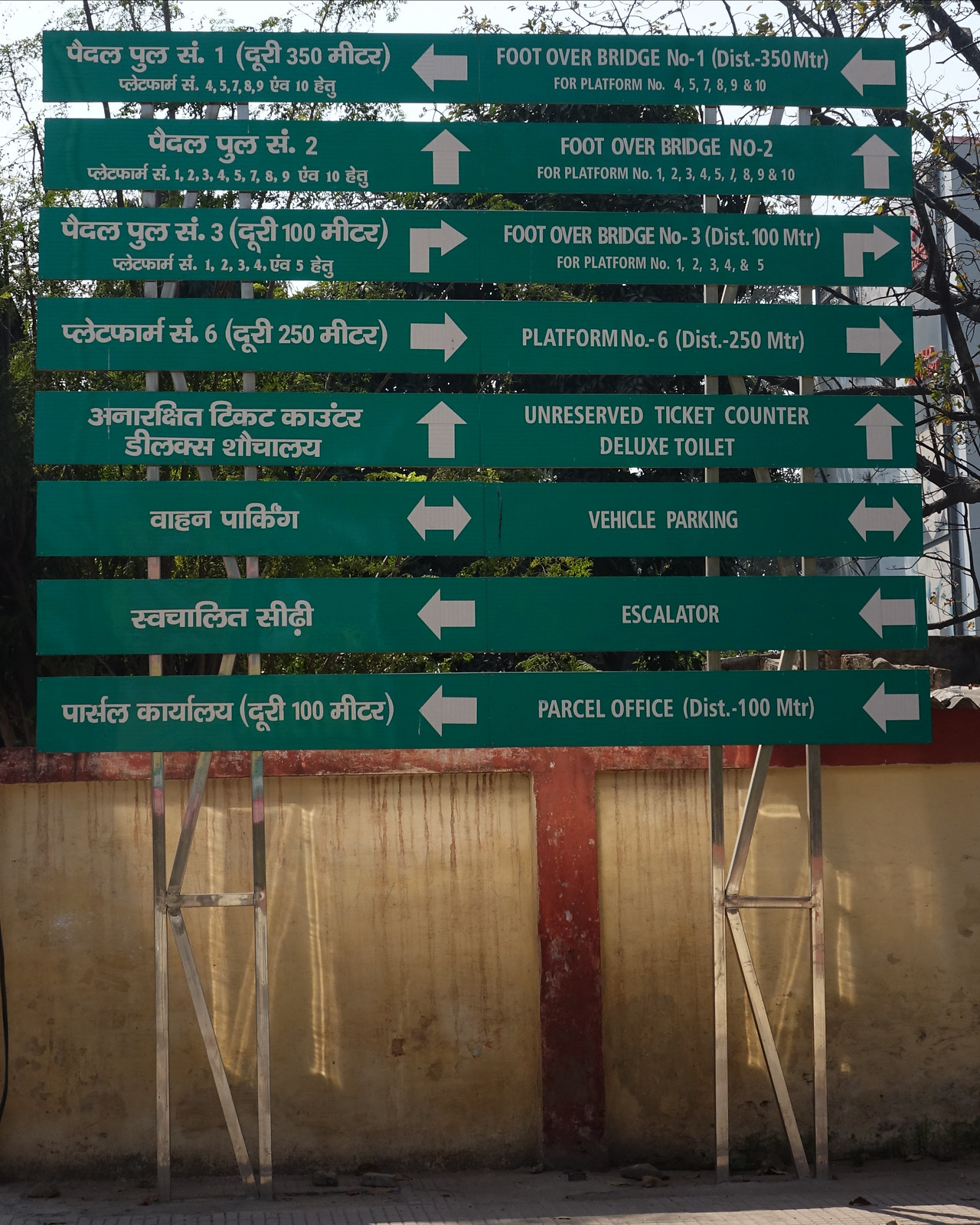The outdoor image is a color photograph depicting a series of eight horizontally stacked green directional plaques or street signs. These signs are mounted on metal posts in front of a worn stone wall adorned with wooden trim. Behind the signs, lush foliage is visible, along with a building situated to the right side.

Each sign is long and slate dark green, featuring text in two languages. The left side, likely in Hindi, and the right side in English, provide identical information with arrows pointing in various directions such as left, right, up, or both left and right. The English text on these signs directs to locations like "foot over bridge number two for platforms 1 through 10," "foot over bridge number three, distance 100 meters for platforms 1 through 5," "platform number six, distance 250 meters," "unreserved ticket counter," "deluxe toilet," "vehicle parking," "escalator," and "parcel office, distance 100 meters." Each sign is supported by triangular columns, with slight gaps between them, creating an organized, easy-to-follow guide to various amenities and directions.